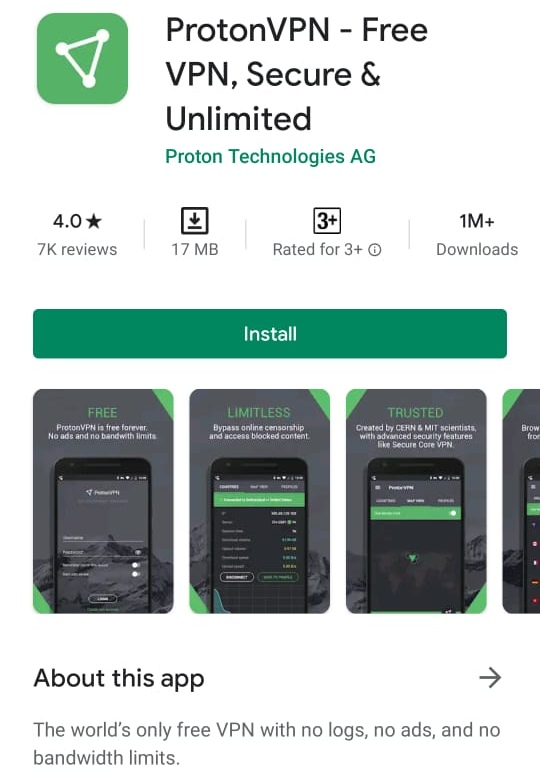This image showcases a detailed screenshot of the ProtonVPN application listing on the Google Play Store. The prominent green square icon features a white, three-pointed triangle with points directed to the left, right, and bottom. Positioned beside the icon is bold, black text that reads "ProtonVPN" with distinctive capitalization for the 'P' and 'VPN'. Following this, is the title "ProtonVPN - Free VPN, Secure and Unlimited", where 'Free VPN' and 'Secure and Unlimited' have varying capitalizations.

Directly below the app title, in green text, is the developer's name, "Proton Technologies AG", with "Proton" distinctly spelled out. The screenshot also highlights the review tab where the app is rated 4.0 out of 5 stars based on 7,000 reviews. There is an icon that signifies the download size of 17 MB. Another icon indicates the app's rating of 3+, meaning it is suitable for users aged 3 and above, and there is a "zero with an i" symbol likely denoting content classification.

On the right side, separated by thin gray bars, it shows the app has been downloaded 1 million times with a "1M+" label, and below it states "downloads" in gray. A dark green rectangle with white text inscribed in the center reads "Install".

Following this, a series of mock-ups display the app in use on various smartphone screens, each snapshot carrying a distinctive label: "Free" highlighted in green, "Limitless", and "Trusted". Adjacent to these images, bold black text reads "About this app". Next to it, a bold gray arrow points to the right, leading into the app's description in regular black text that proudly declares, "The world's only free VPN with no logs, no ads, and no bandwidth limits."